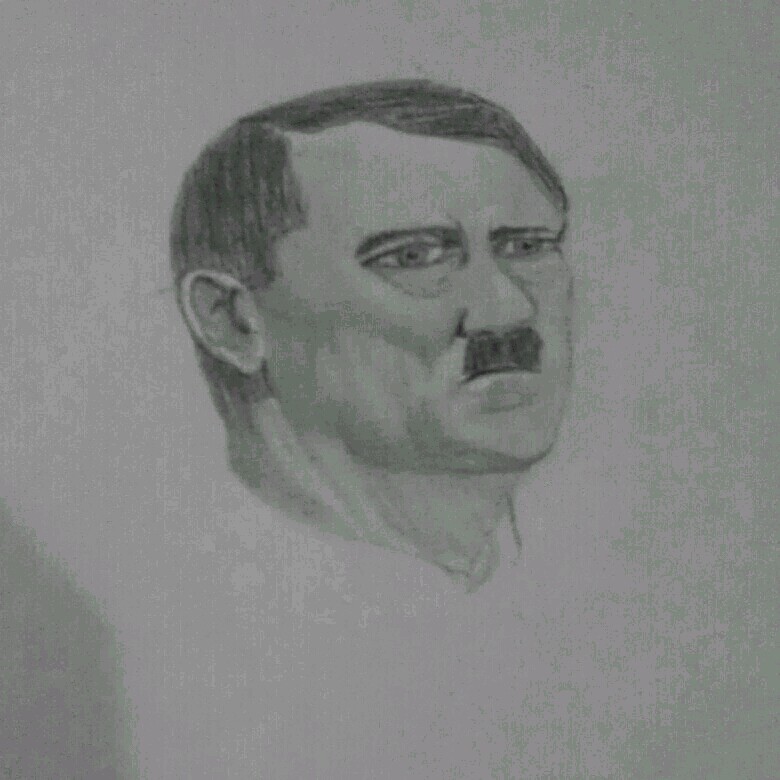In this image, there is a meticulously detailed drawing executed in black pencil on medium grayish paper with hints of green. The subject is a head-and-shoulders portrait of a man strongly resembling Adolf Hitler, facing slightly towards the right in a three-quarter view. The man's characteristic small mustache, situated just below each nostril, and the distinctly parted and dark-shaded hair typical of Hitler are finely rendered. The face and neck are shaded in blue, adding a monochromatic depth, while the hair and mustache are heavily shaded in black. The left ear, visible due to the angle, is carefully detailed, as are the deep-set eyes with black pupils against white sclera, and the bags under the eyes that convey a sense of realism. The drawing skillfully captures the contours of the man's cheeks, the stout appearance of his face, and the fine shading of the neck, which is cut off at the bottom of the image. A subtle shadow extends from the bottom left, adding to the three-dimensional effect of the portrait.